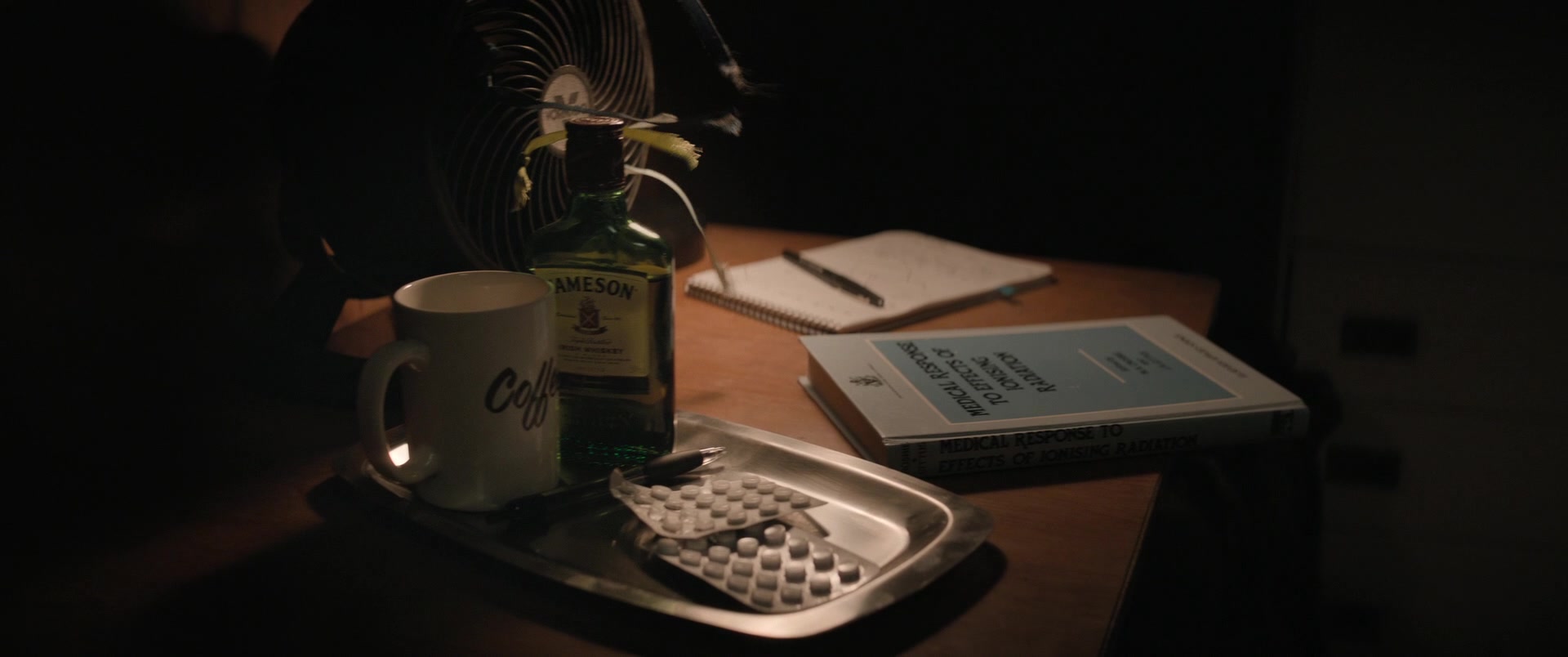Amidst a dimly lit setting with a dark backdrop, a brownish wood grain desk or countertop serves as the stage for an array of items. Dominating the center, a spiral notebook lies horizontally with a pen resting across its open pages. Just below this notebook, a hardcover book with a light blue cover adds a touch of color to the scene. To the left, a silver serving tray holds two sheets of blister-pack pills. Flanking this setup, on the right, sits a pristine white coffee mug. Completing the vignette, a fifth-size bottle of Jameson whiskey stands sentinel to the right of the coffee mug. The arrangement is bathed in subtle darkness, offering a glimpse into a moment paused in subdued lighting.